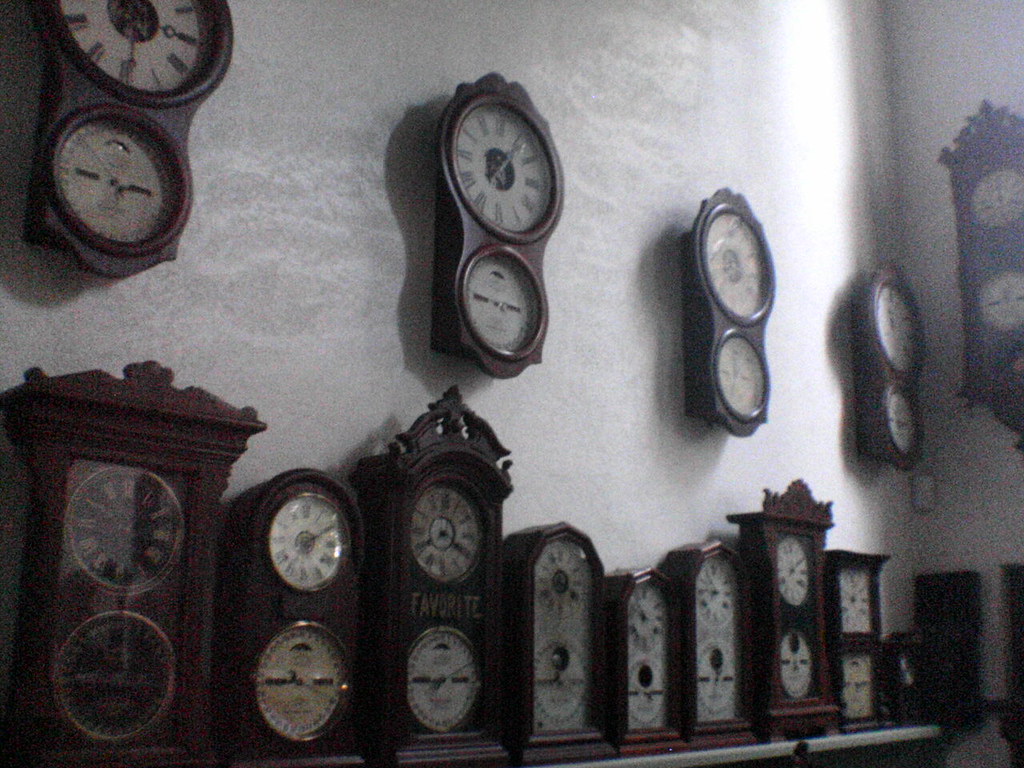The image showcases a light gray or white wall adorned with a collection of intricately designed small grandfather-style clocks. The wall features five prominent double-faced clocks, each with a larger clock face on top displaying Roman numerals and a smaller, circular thermometer face below. These clocks are set in elegant dark brown wooden frames, some with smooth rounded tops and others with pointed decorative borders. Below these, a wooden shelf holds a line of ten additional double-faced clocks. These clocks vary in design, with some showcasing black faces with gold numbers and others having white faces with black numbers. Each clock and thermometer pairing is distinctly styled, contributing to the ornate and diverse display. The image, likely taken in a clock shop, cuts off slightly, hinting at more clock designs around a visible corner on the right side wall.